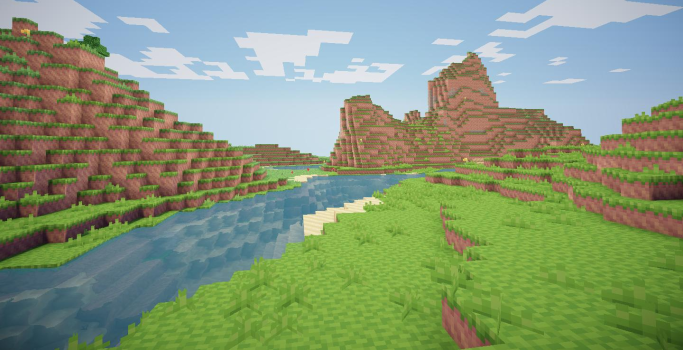This is a color photograph of a computer game with blocky and primitive graphics, reminiscent of early console games. The image features a blue sky at the top, interspersed with blocky, greyish clouds. On the left side, there is a blocky hill or mountain composed of brown blocks, topped with a layer of green grass. Below, a green grass ledge runs horizontally, leading into a river that flows from the lower left corner towards the center of the image. The river appears blocky, flanked by white blocks at its center.

In the foreground, towards the right, there are patches of blocky grass and small shrubs. The scene also features a series of wide steps covered in grass, narrowing slightly towards the right. The background is dominated by rocky mountains or cliffs with intermittent patches of grass, adding depth to the image. The overall composition evokes the nostalgic charm of early video game landscapes.